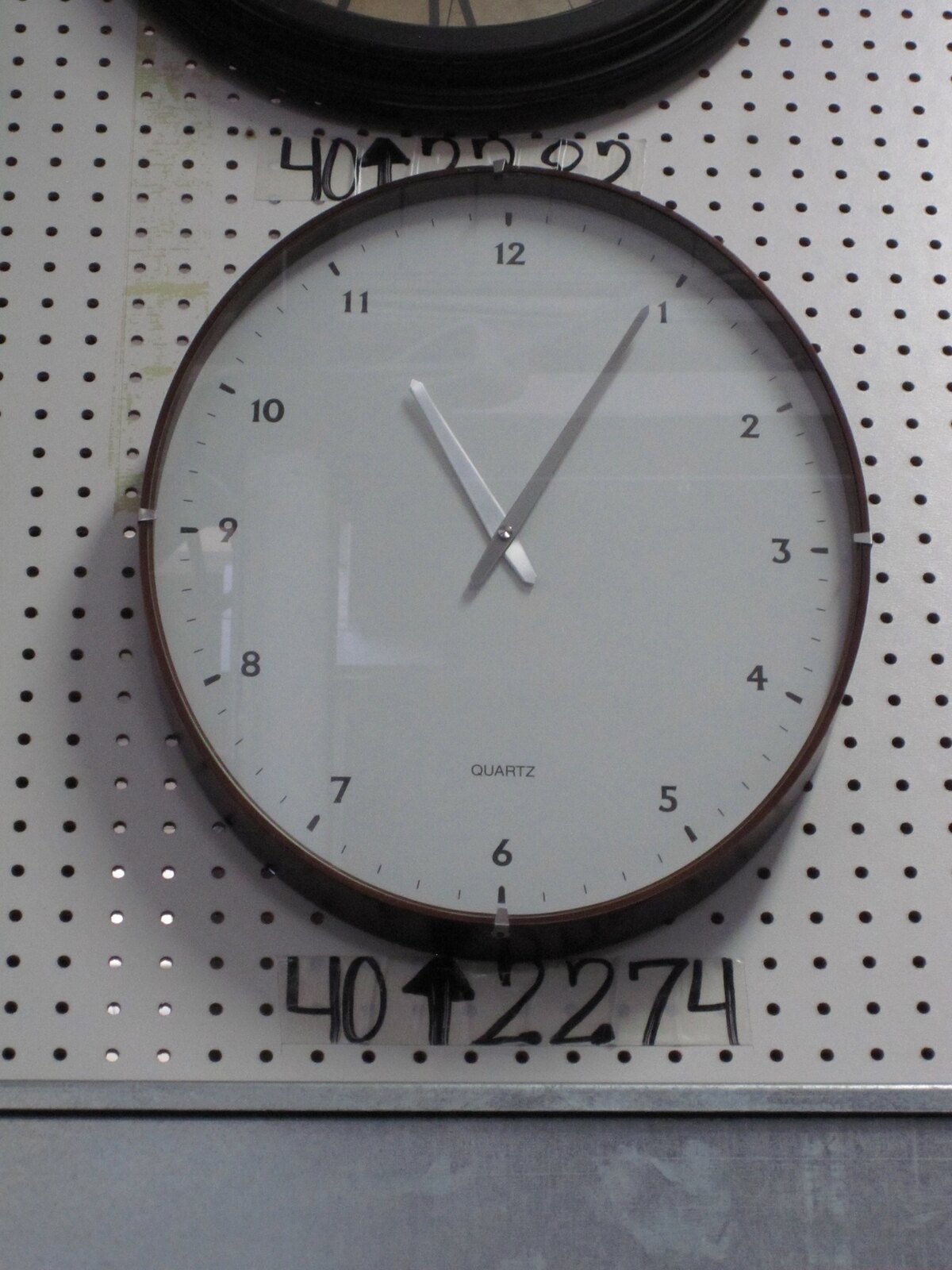The image features a wall adorned with multiple clocks, each distinctly labeled with specific numbers. The primary clock, prominently displayed, shows the number "40" accompanied by an upwards arrow and the number "2274," all written in black marker on a pegboard. Positioned above this clock is another clock partially visible, labeled "40" with an upwards arrow and what appears to be "2282," though it is partially obscured by the main clock. The main clock itself is encased in a black-trimmed circle with a glass cover. Its silver hour and minute hands display the time as 11:04, nearly 11:05. Notably, this clock lacks a second hand and is identified as a quartz model, seemingly used to indicate time for a specific region as part of an organized display.